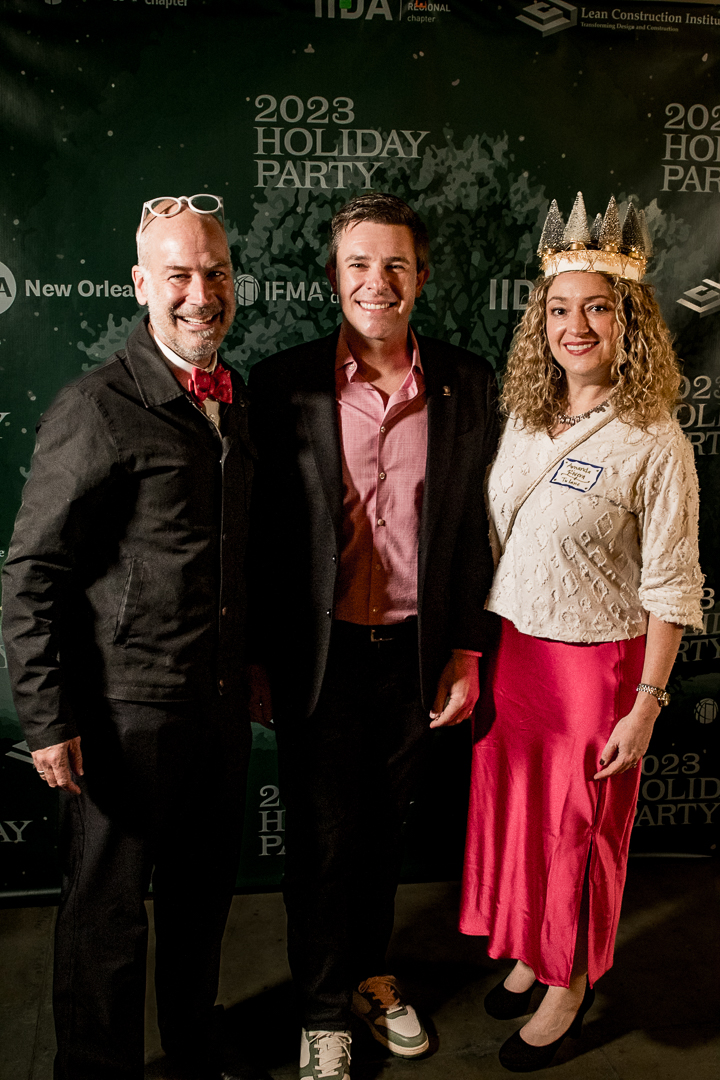The photo captures three smiling individuals standing in front of a festive backdrop that reads "2023 Holiday Party." The man on the left, who is bald, is wearing white-rimmed glasses perched on his forehead, a red bow tie, a black jacket, and black pants. The man in the middle, with short, gelled brown hair, is dressed in a black sports coat, red shirt, black pants, and white sneakers. The woman on the right, crowned and adorned with a necklace, has shoulder-length curly hair, a red dress paired with a white top, and a paper name tag on her chest. The background banner features the text "New Orleans" on the left, "IFMA" in the middle, and "IID" on the right, adding to the celebratory atmosphere of the event.